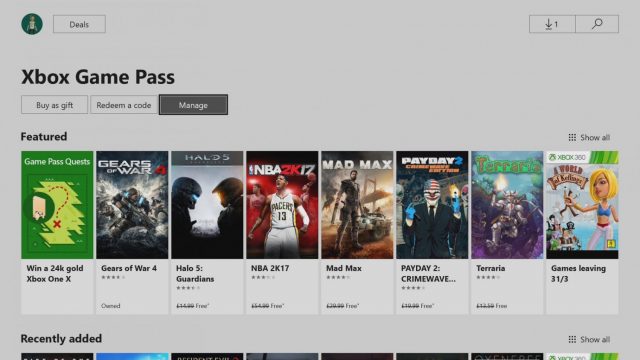This detailed image shows a screenshot of the Xbox Game Pass interface. The background is visually appealing, enhancing the overall aesthetic. At the top, there is a distinctive green circle with an eye beside it, followed by a rectangular box labeled "DEALS." To the right, another rectangular box features a downwards arrow indicating the download icon, next to the search icon.

Prominently displayed in bold black letters is the text "XBOX GAME PASS." Below this, there are three interactive buttons: "BUY AS GIFT," "REDEEM WITH CODE," and "MANAGE." The "MANAGE" button stands out as it is highlighted with a black background and white letters.

The middle section is labeled "FEATURED" in black letters. This area showcases a selection of game posters. The first poster advertises a chance to "WIN A 24 KG XBOX ONE X." Following this are posters for various games including "GEARS OF WAR 4," "HALO 5," "NBA 2K17," "Mad Max," "Payday 2," and "Terraria," plus a "Games Leaving" poster. In total, there are seven featured posters displayed.

At the bottom of the visible screenshot is the heading "RECENTLY ADDED," although the images beneath this section are cut off and not visible.